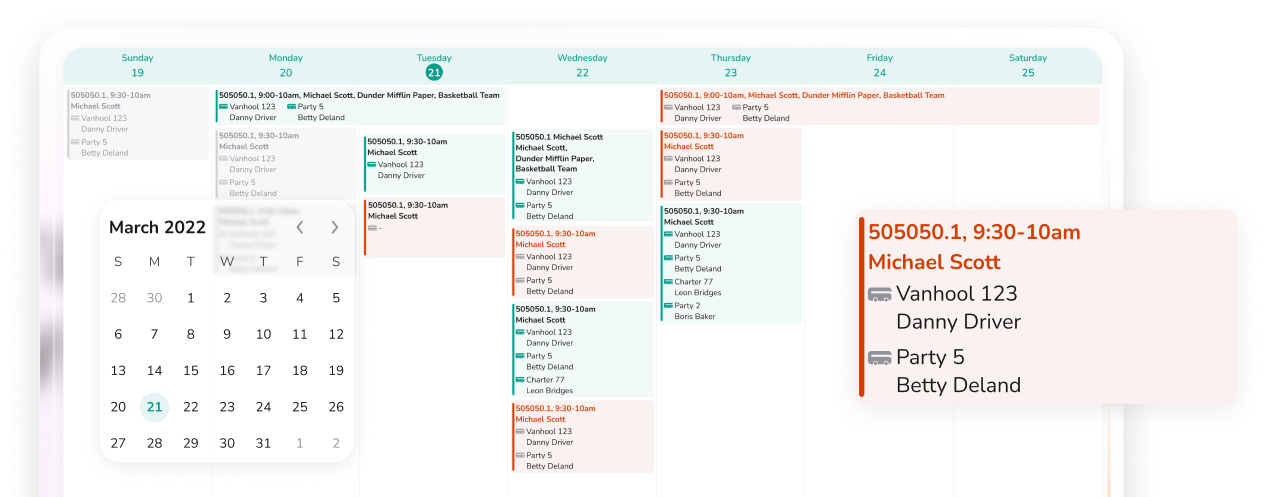The image depicts a detailed interface of a calendar or scheduling application. The upper section of the app displays a week view, with each day of the week labeled: Sunday through Saturday. Each day is marked with a distinct number, such as "1900" for Sunday, "2000" for Monday, progressively increasing to "2500" for Saturday. Below this top portion, there are various entries indicating events scheduled throughout the week, some of which overlap in time across multiple days.

One card in the middle of the interface appears to be selected or edited, showing a pop-up for the month of March 2022 with the 21st highlighted, suggesting the editing of an event date. Each calendar entry is accompanied by details such as start and end times, indicated by numbers preceding the dates.

On the right side of the app, there is another detailed pop-out section displaying additional event information. This section lists specific time slots, such as 9:30 AM to 10:00 AM, along with the names "Michael Scott," "VanHoo123," and "Danny Driver." Below this, another entry lists "Party5" and "Betty Deland," hinting at possible reservations.

The overall design and details suggest that this application might serve as both a scheduling and reservation tool, organizing multiple user entries and providing comprehensive date and event management features.